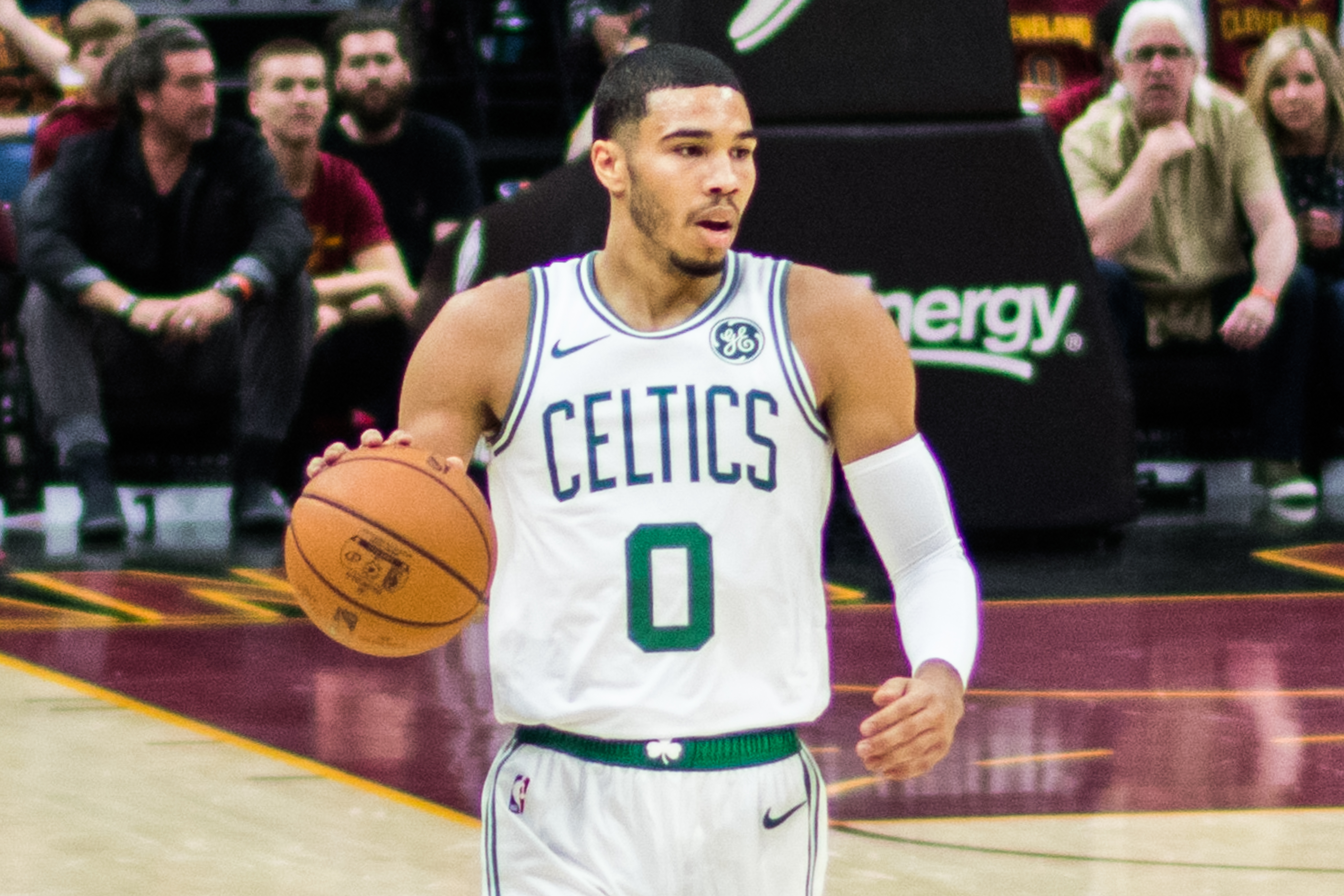In the image, a professional basketball player from the Boston Celtics, identified as Jason Tatum, is captured mid-game as he dribbles a basketball with his right hand. Tatum, a Black man with a short haircut, a scruffy beard, and a closely shaved goatee, is prominently wearing a white tank top with green accents, emblazoned with the word "Celtics" across the chest and the number zero on his jersey. His white shorts feature red pinstriping down the sides.

The setting is a basketball court with a distinctive maroon and yellow color scheme on the floor. Behind Tatum, the bottom half of a basketball hoop is visible, featuring a base with the word "Energy" in the background, possibly indicating a sponsor. The viewer also sees an audience seated on the sidelines, with some fans wearing black, red, and tan clothing. To the upper right, a man dressed in a black shirt and black pants sits with his hands folded. Nearby, another man in a red shirt and young spectators surround him. In the upper left corner, more spectators can be seen, including a man with white hair resting his hand on his chin and a lady next to him. The vibrant scene captures the intensity and atmosphere of a professional basketball game.